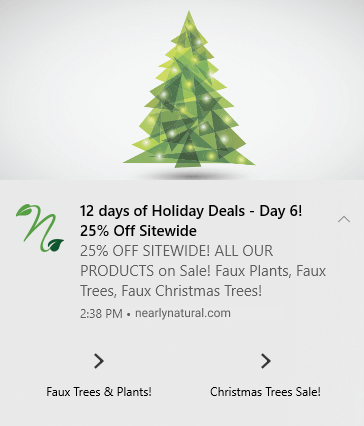This is a detailed description of an illustration featuring a promotional advertisement. The image is a grainy, upright, gray rectangle divided into two main sections.

In the top half of the gray rectangle, there is a whimsical depiction of a Christmas tree that appears to be floating due to the shadow cast below it. Notably, this tree lacks a visible trunk or stem, enhancing the illusion of it hovering in mid-air. The Christmas tree is constructed from a series of overlapping, transparent triangles in varying shades of light and dark green. At the peak of the tree, where an ornament is traditionally placed, the shapes converge, standing upright. Scattered within the triangular shapes are white dots, resembling festive lights.

The bottom half of the gray rectangle features black text and numbers, beginning from the middle of the section and continuing downward. The text reads, "12 days of holiday deals - Date: 6! 25% off statewide, 25% off statewide. All our products are on sale: faux plants, faux trees, faux Christmas trees! 2:38 p.m. yearlypicture.com." Additionally, in the lower right corner of this gray rectangle, there are two arrows pointing to the right. One arrow is labeled "faux trees and plants," and the other is labeled "Christmas tree and sale."

This detailed promotional image effectively combines a festive visual with clear, informative text to attract attention and convey the message of holiday sales.